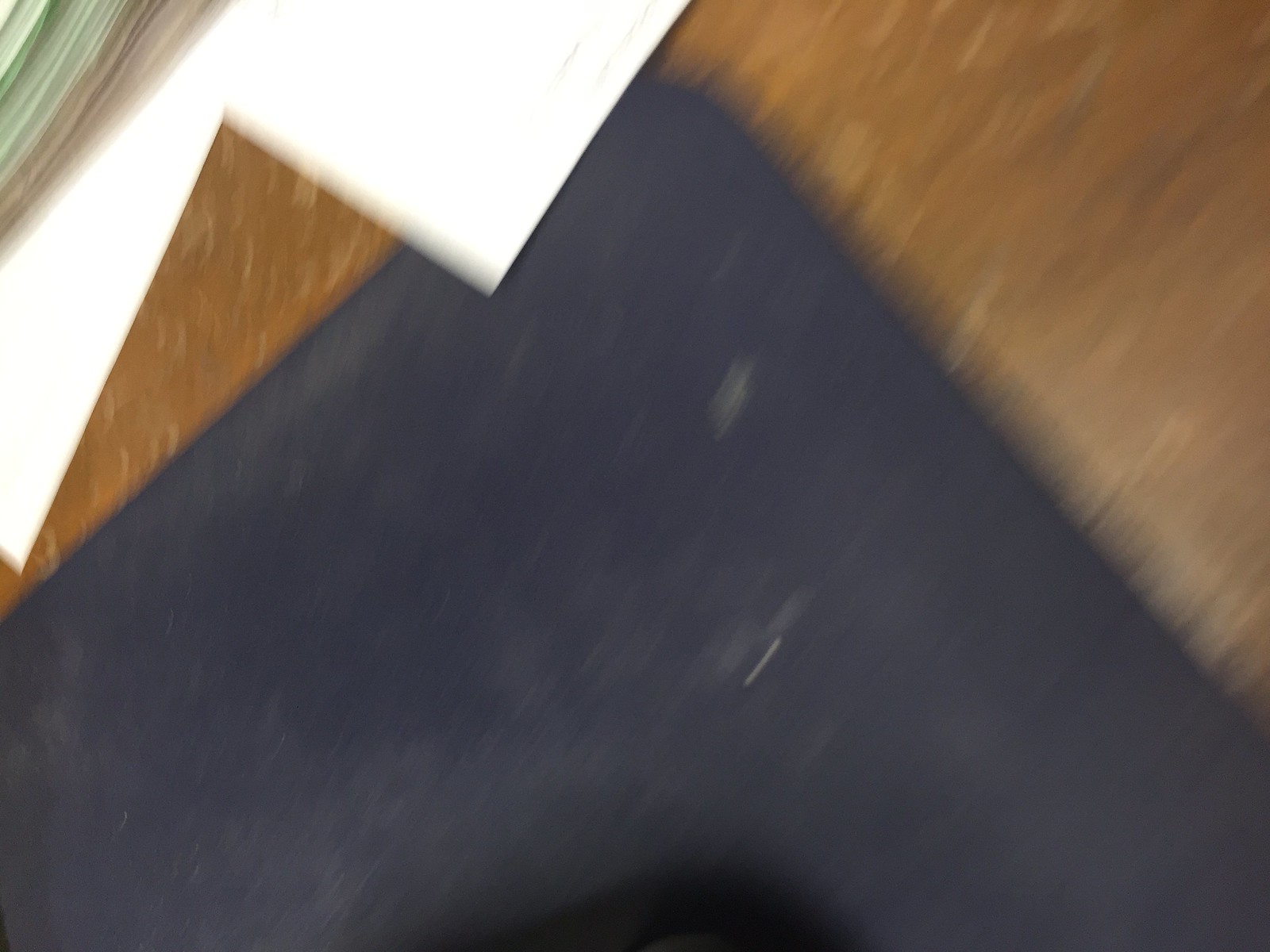This color photograph is a close-up image that is somewhat blurred, making it challenging to distinguish the objects clearly. In the upper left-hand corner, a series of light and dark green stripes are visible, followed by beige stripes just below them. Dominating the center of the image is what appears to be the edge of a large black object, possibly a placemat or tray, with noticeable scratches - some blurred, one more in focus - in the middle. At the bottom edge, there is a near-triangular dark shadow. The black object is set on a wooden surface that shows visible wood grain textures. Towards the left, a distinct brown wooden triangle can be seen, while the upper right-hand corner features a larger, more blurred triangle of wood grain with lighter flecks interspersed. Additionally, some paper or white objects are barely visible at the top of the brown surface, positioned towards the center and left.